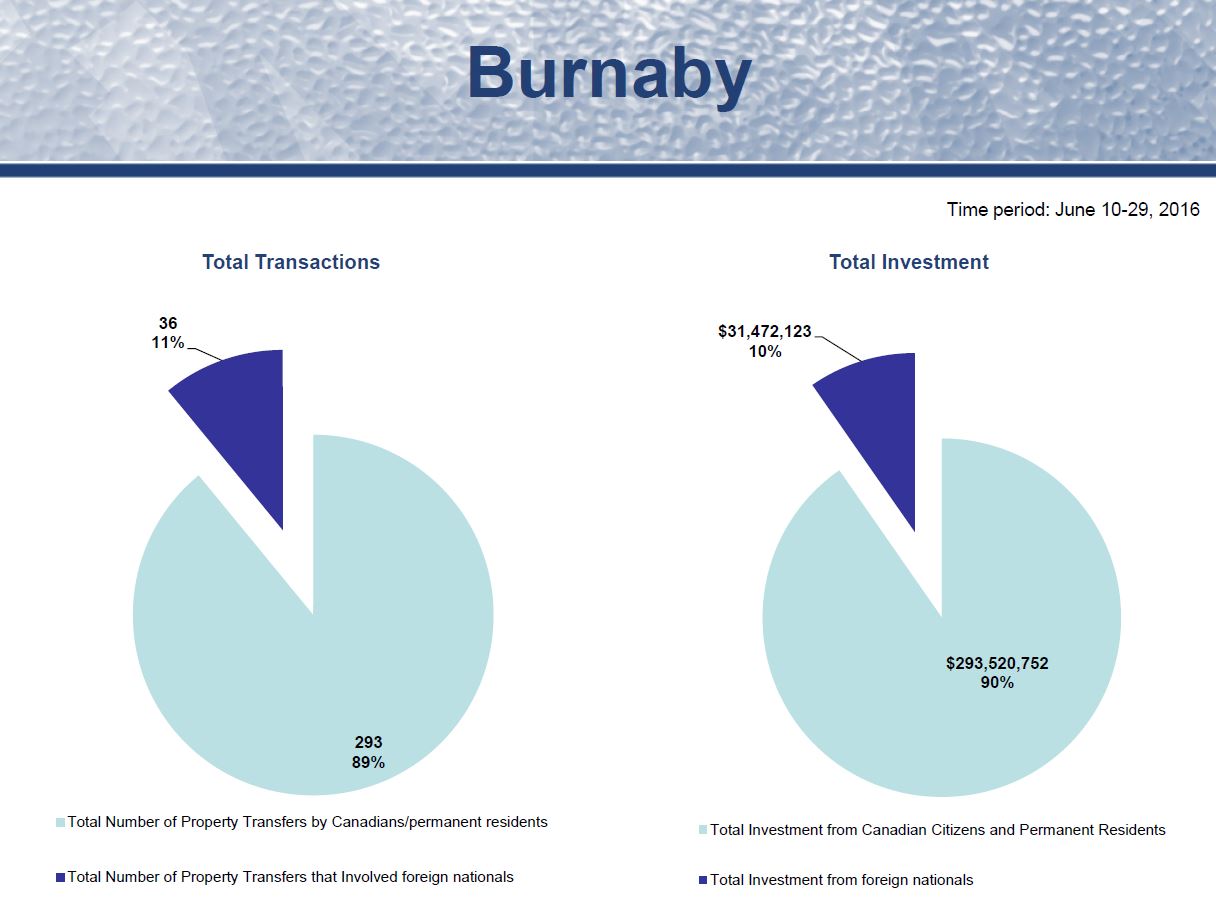The image titled "Burnaby" prominently features two pie charts detailing property transactions and investments for the period around June 10, 2016. The left pie chart illustrates the total transactions involving property transfers. The lighter blue section, making up 89%, indicates transfers by Canadians and permanent residents with 293 transactions, while the darker blue section, 11%, represents 36 transactions involving foreign nationals. The right pie chart depicts total investments, where the light blue, constituting 90%, represents $293,520,752 from Canadian citizens and permanent residents, and the dark blue, 10%, signifies $331,472,123 from foreign nationals. These pie charts collectively provide a comparative visual breakdown of local and foreign participation in Burnaby's property market during this period.